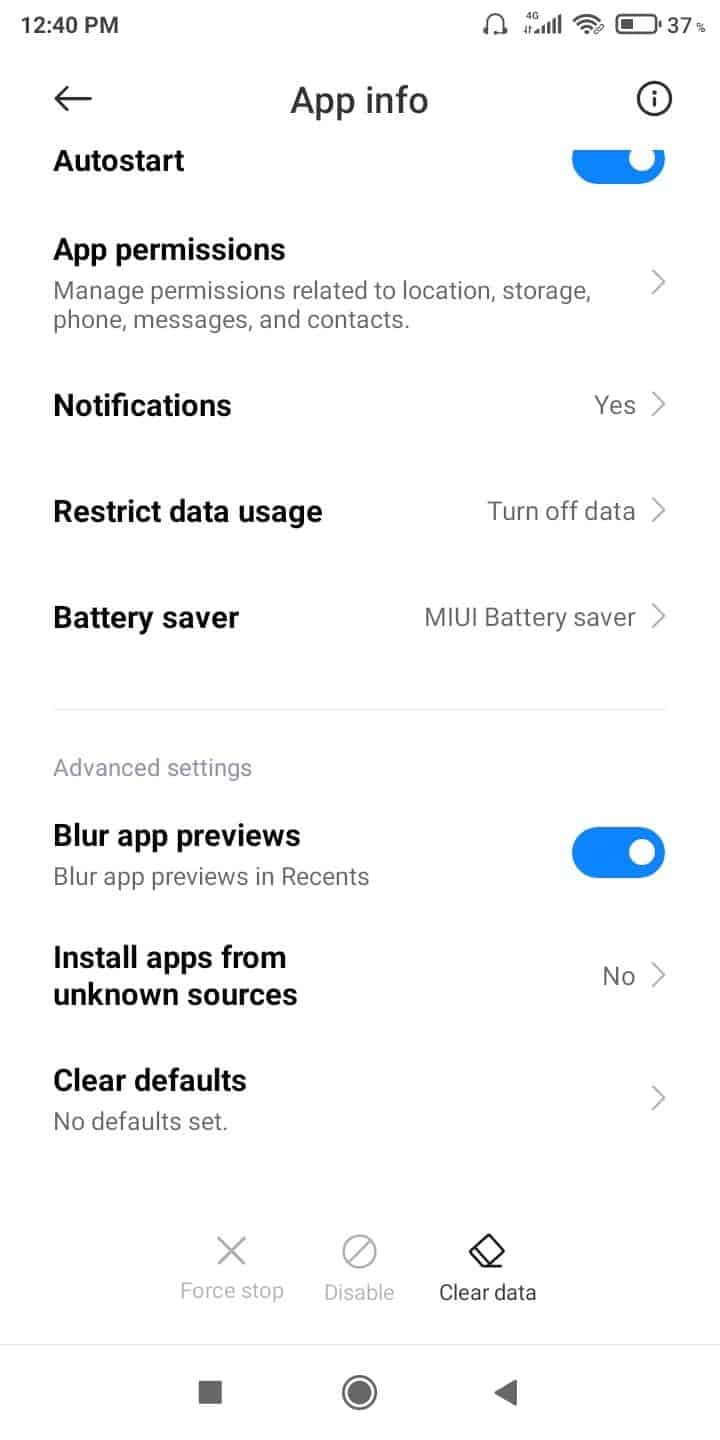A detailed caption for the image could be:

---

This image captures a close-up of a mobile phone screen displaying the "App Info" page. The interface begins with a section titled "Auto Start," accompanied by a blue toggle switch indicating it is enabled; the white toggle is positioned on the right. Directly below, in black text, is "App Permissions," followed by a gray subtext outlining the management of permissions related to location, storage, phone, messages, and contacts. The next visible item is "Notifications," which indicates "Yes" beside it in black text. Further down, "Restrict Data Usage" appears with an option to "Turn off data." Following this section, there is a battery management setting labeled "Battery Saver," specifically the "MIUI battery saver" mode. A faint gray line provides a visual divider before entering the second section of settings. At the bottom of the first section, "Advanced Settings" is mentioned in gray text. In the subsequent section, "Blur App Previews" is noted in black text, with a gray subtext explaining its functionality to "blur app previews in Recent.” The setting is shown to be active, illustrated by a blue slider with a white dot on the right side. The page continues with additional settings that extend beyond the captured portion of the screen.

---